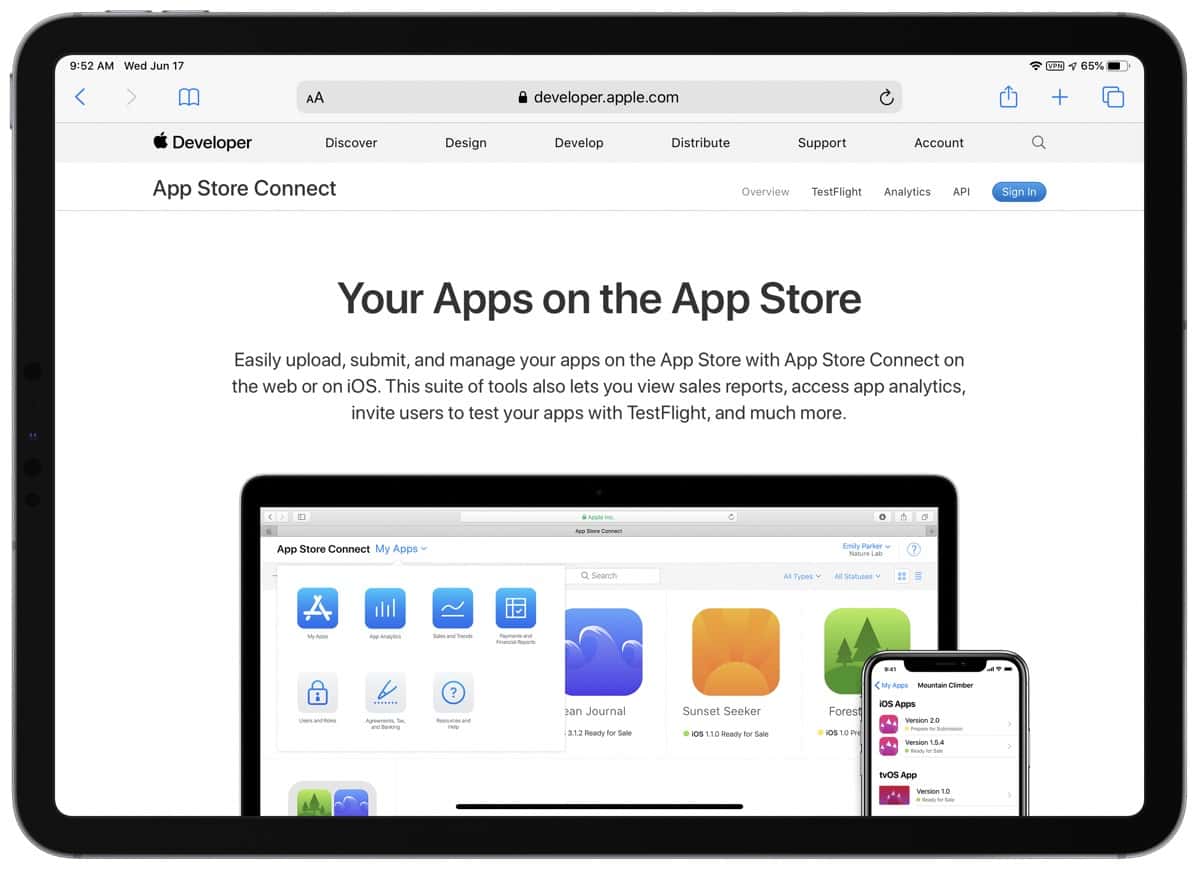A detailed image caption:

The image showcases a tablet screen, where the edges of the tablet are visible. The top of the screen displays the current time, 9:52 a.m., and the date, Wednesday, June 17. To the right, there's an icon showing Wi-Fi connectivity, and the battery indicator reads 65%. Below the status bar is a search bar with the URL "developer.apple.com" entered. Beneath the search bar is a navigation menu with options: Discover, Design, Develop, Distribute, Support, and Account. 

Further down, the screen presents another navigation bar with sections labeled: Overview, TestFlight, Analytics, API, and Sign In under the heading, "Apple Store Connect." Below, the text reads: "Your apps on the App Store. Easily upload, submit, and manage your apps on the App Store with App Store Connect on the web or iOS. The suite of tools also lets you view sales reports, access app analytics, invite users to test your apps with TestFlight, and much more."

The image also includes a visual representation of a tablet and a phone, both with black edges and white backgrounds, adding to the theme of viewing devices on another digital device. The overall background remains predominantly white with vibrant accents of purple, blue, orange, green, and pink, enhancing the visual appeal.